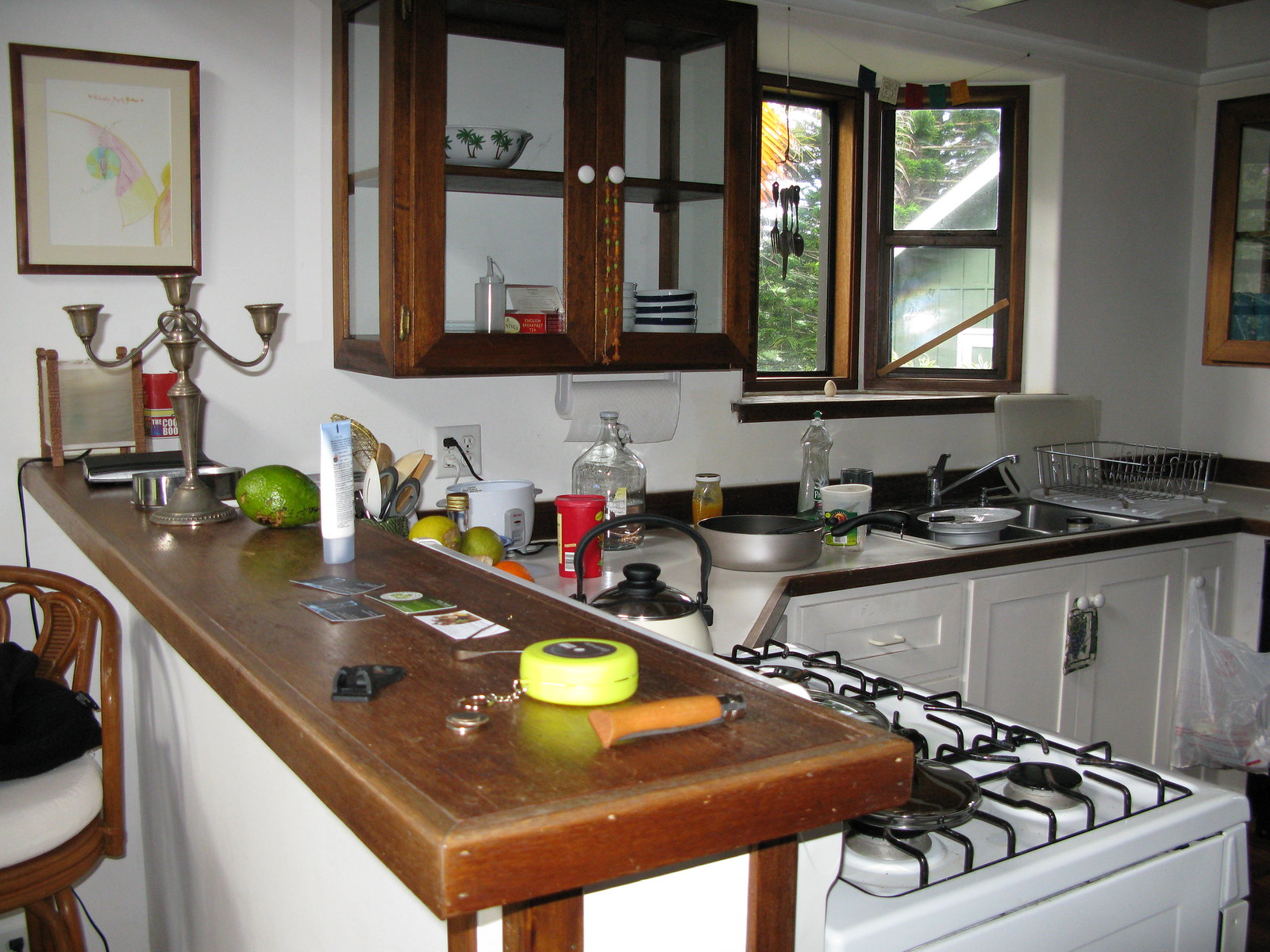This color photograph captures a detailed view of a cozy kitchen. On the left side, a wooden bar extends from the countertop, creating a higher seating area designed for high bar stools. The bar top is adorned with a variety of items including a tarnished silver candelabra, a green avocado, a tube of cream, a collection of business cards, a lime green round canister, and a yellow lighter. Beneath the bar, a wooden bar stool with a white cushion is tucked in neatly.

The kitchen features white walls and is dominated by a white color scheme. The countertops, cabinets, and lower cabinets are all pristine white. A white gas stove sits on the kitchen side of the bar, topped with a white tea kettle. The sink area boasts a double basin stainless steel design, complemented by a polished chrome faucet. A stainless steel dish rack is positioned next to the sink for drying dishes.

Above the sink, a wooden frame window enhances the space with natural light and decorative charm, featuring a hanging wooden chime. To the left of the sink, against the wall, there is an additional cabinet with a wooden frame and clear glass panels, providing extra storage and a touch of elegance to the kitchen's decor.